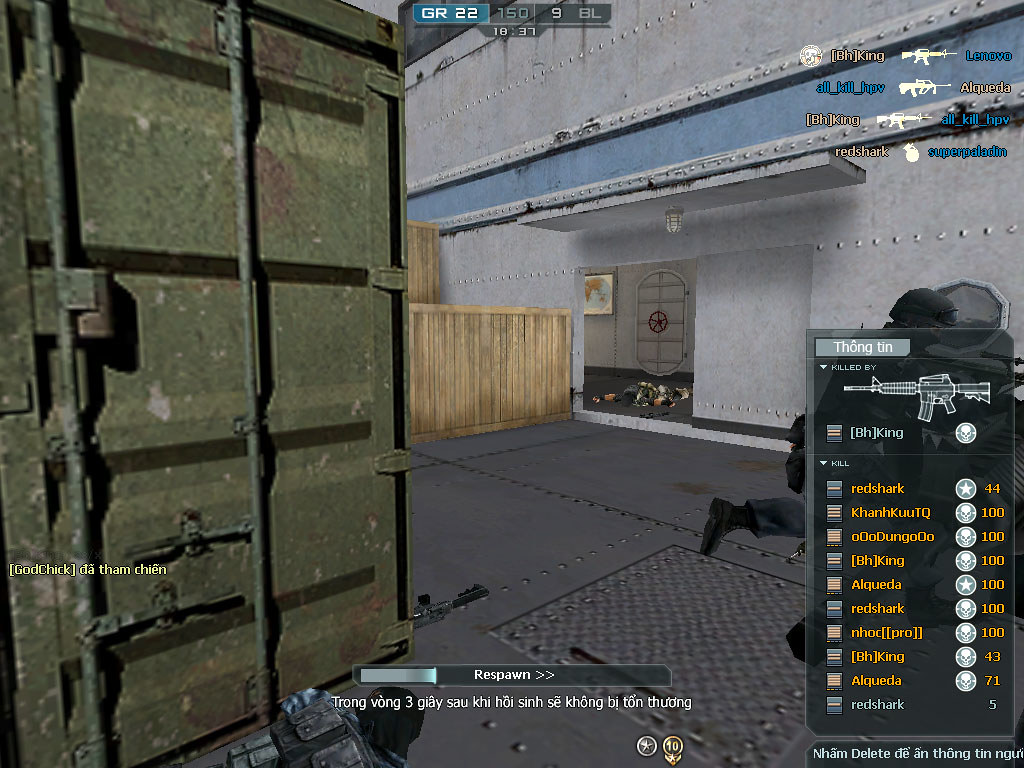In this screenshot from a first-person shooter video game set in Vietnam, which heavily resembles the classic "Goldeneye" game, the interface displays various game elements predominantly in Vietnamese. In the lower right, there is a gun class selection featuring multiple firearms, with a noticeable option labeled GR-22-159-BL-ATTACK. The scene includes interactive features such as a black gate adorned with metal elements and a wooden crate, emphasizing the detailed environmental design that players can navigate. The gameplay setting appears to be within a ship or industrial facility, highlighted by a green shipping container in the foreground and what looks like a ship hull in the background. The upper right corner showcases a list of players, potentially from multiple teams, with names such as King, All-Kill, Red Shark, Lenovo, Al-Quaeda, and Super Paladin, indicating the competitive nature of the match. The image encapsulates the dynamic and immersive elements characteristic of a multiplayer shooter experience, enriched with respawn capabilities and strategic gameplay.